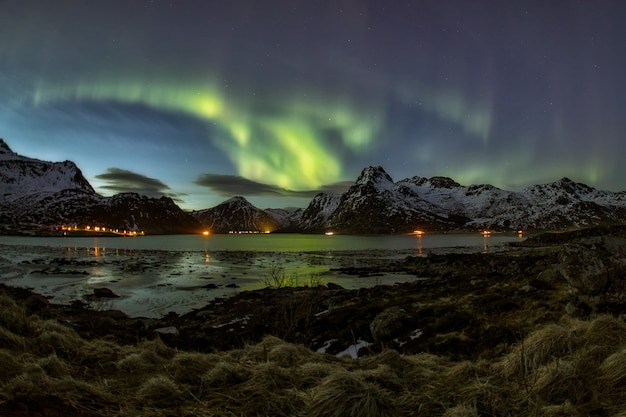The serene photograph captures a breathtaking nighttime landscape in the Northern Hemisphere, showcasing the awe-inspiring Aurora Borealis stretching across a deep midnight blue sky. Snow-capped mountains form a majestic silhouette against the celestial display, with patches of green aurora illuminating the dark surroundings. In the foreground, a rugged terrain of bushes, rocks, and patchy grass leads to the edge of a reflective body of water, possibly a frozen lake. Mirroring the vibrant lights of the aurora, this water adds to the ethereal beauty of the scene. The base of the mountains is dotted with clusters of orange lights, suggesting small towns or campsites, adding a cozy element to the otherwise expansive, wild landscape. The absence of text allows the natural splendor to speak for itself, making the entire scene appear both peaceful and grandiose.